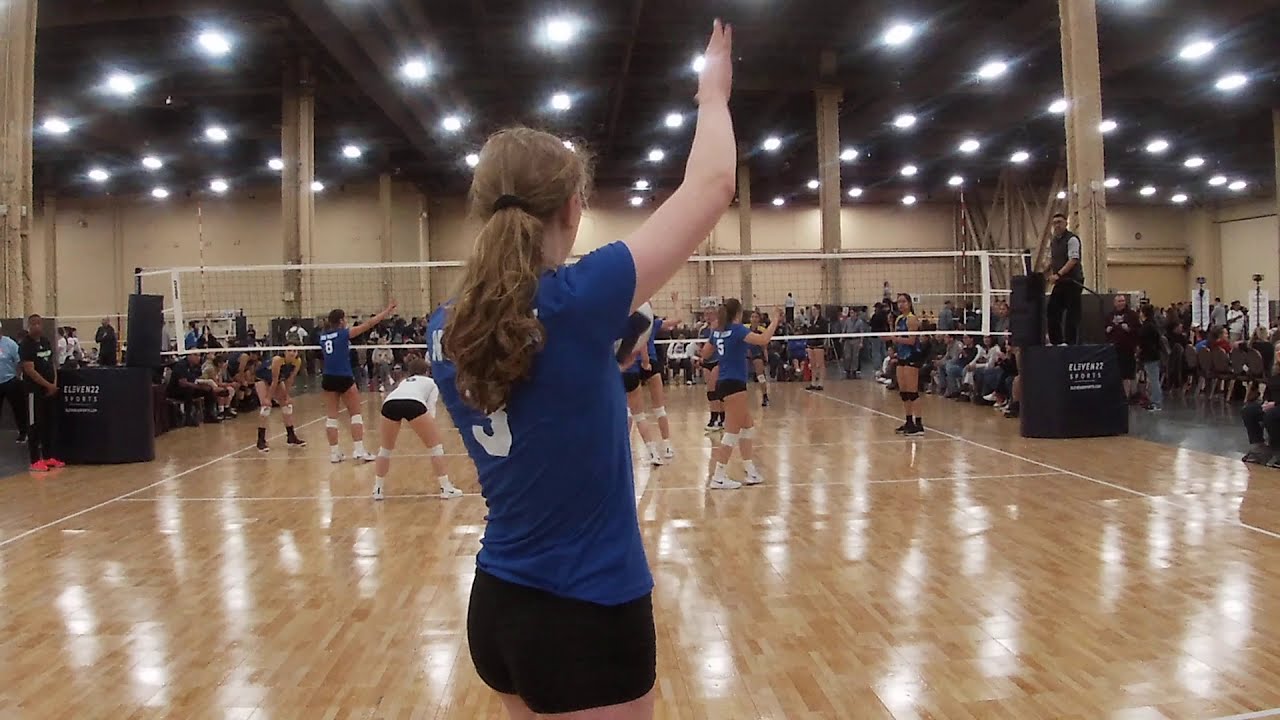The horizontally-aligned rectangular photo captures an intense moment inside a gym during a girls' volleyball game. Dominating the foreground is the backside of a young girl, poised to serve. She has long brown hair pulled into a ponytail and is dressed in a blue t-shirt featuring a white number—likely a 3, though partially obscured by her hair—and short black shorts. Her right arm is raised, ready to serve the ball she holds in her left hand. The middle of the image is bisected by a volleyball net, stretching from left to right, with players on either side prepared for the serve. Both teams wear knee pads and white tennis shoes; the team in the foreground sports blue jerseys with white text, while the libero stands out in white. The opposing team, further in the background, appears clad in darker gray or black tops. Spectators sit and stand along the sides of the gym, which has light brown walls. On a raised platform near the net, a referee in a black vest, short-sleeved shirt, and black pants closely watches the server. The scene vividly captures the anticipation and focus characteristic of a competitive indoor volleyball match.